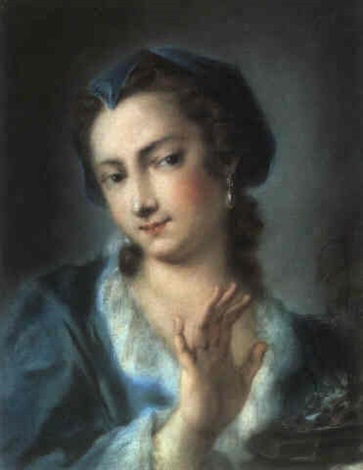This detailed oil painting portrays a young Caucasian woman from the 1700s, depicted from the head and shoulders against a predominantly dark gray wall, which becomes slightly lighter behind her head. Her face is tilted slightly to the left, but her large, dark brown eyes gaze forward, creating a captivating focal point. She has a pointed nose, dark pink lips, and rouged cheeks that add a touch of red to her very fair, white skin.

Her dark brown hair is meticulously pulled back, covering her ears and curling slightly as it reaches the back of her neck. Notably, she possesses a widow's peak with a blue streak or possibly a velvet cap adorning her head, blending into her hair and adding subtle elegance. 

She wears a period costume, primarily dark blue with a detailed white and blue collar and cuffs. The dress is open at the neck with a V-neck style. Completing her attire are large pearl earrings that lie just in front of her hair.

Her right hand is raised with the palm open and fingers slightly spread, including the pinky which is tilted slightly back, as if gesturing 'stop' to the viewer. This poised and detailed gesture, along with her steady gaze, adds depth and intrigue to the portrait.